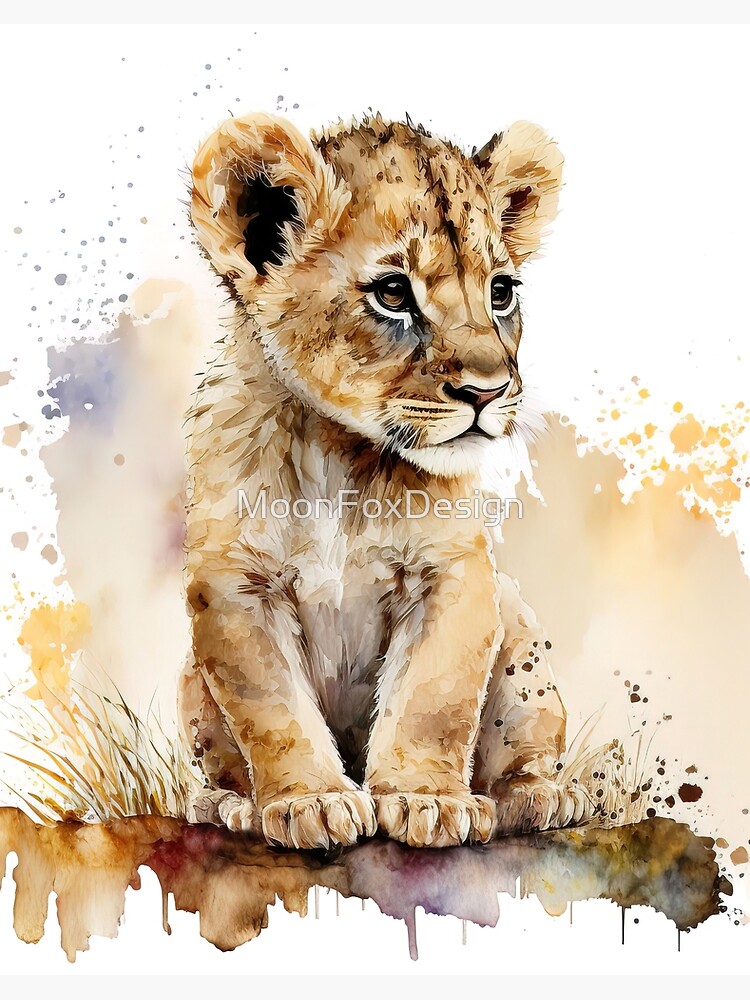This image, titled "Moon Fox Design," showcases a digitally crafted watercolor depiction of an adorable baby lion cub. The cub's body faces forward with his front paws placed closely together, and he gazes off slightly to the right with a touch of curiosity in his eyes. His white belly peeks out between his paws while his fur, detailed in watercolor, gives him a cute and fuzzy appearance. The surface beneath the cub mimics dripping watercolor, reminiscent of a rocky texture in various shades of fresh soil, grass leaves, and wildflowers. The background features an off-white to beige wash that transitions into splatters of orange, blue, and purple hues, creating a vibrant yet serene backdrop. The image is centered with a visible watermark, ensuring its protection against reproduction.